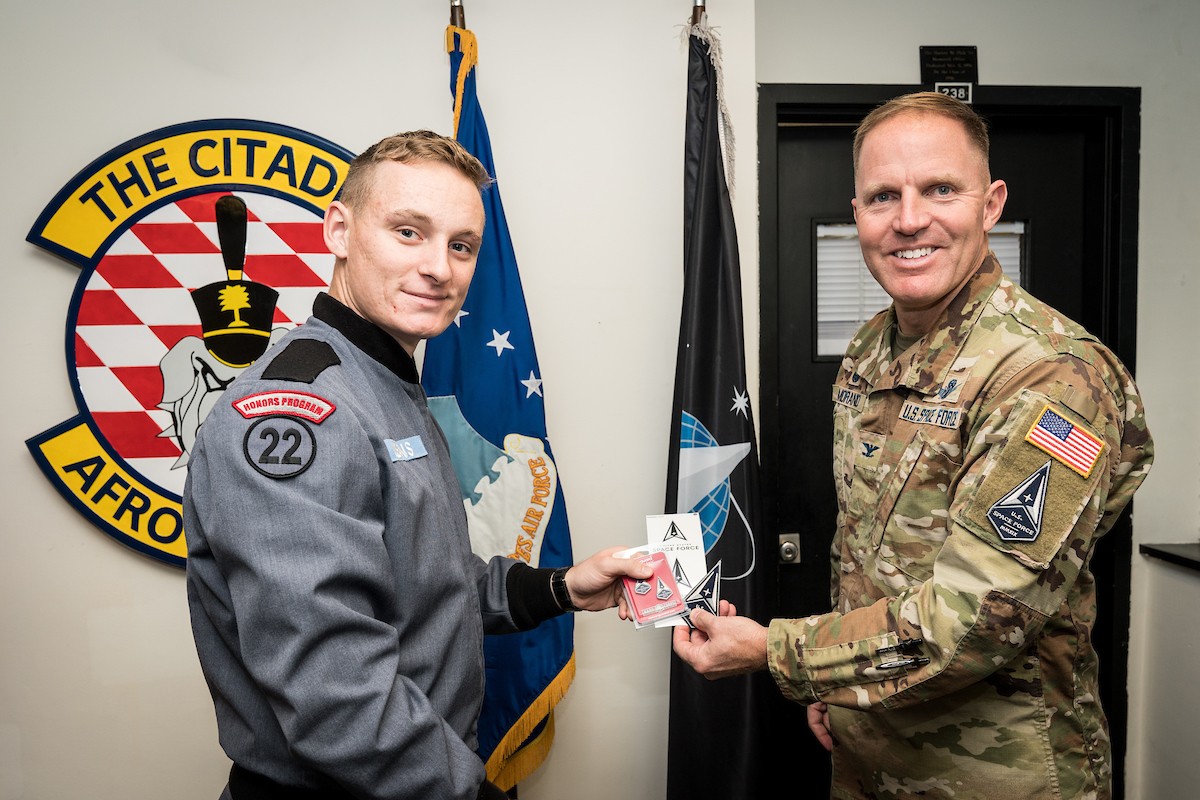In a room with beige walls and a black door, two men are standing in front of a flag and an emblem that reads "The Citadel" and features a bulldog on a red and white checkerboard pattern. One man, wearing a grey outfit adorned with a red and white "Honors Program" patch above a black circle with the number 22, is positioned next to the flag. The other man, dressed in a U.S. Space Force camouflage uniform, stands beside him. Both appear to be in their 30s to 40s, and they are looking at the camera, smiling, and holding various items, possibly badges or stickers, which are red, white, and black with some arrow shapes. The scene likely captures an award ceremony or the exchange of honors in an office setting.